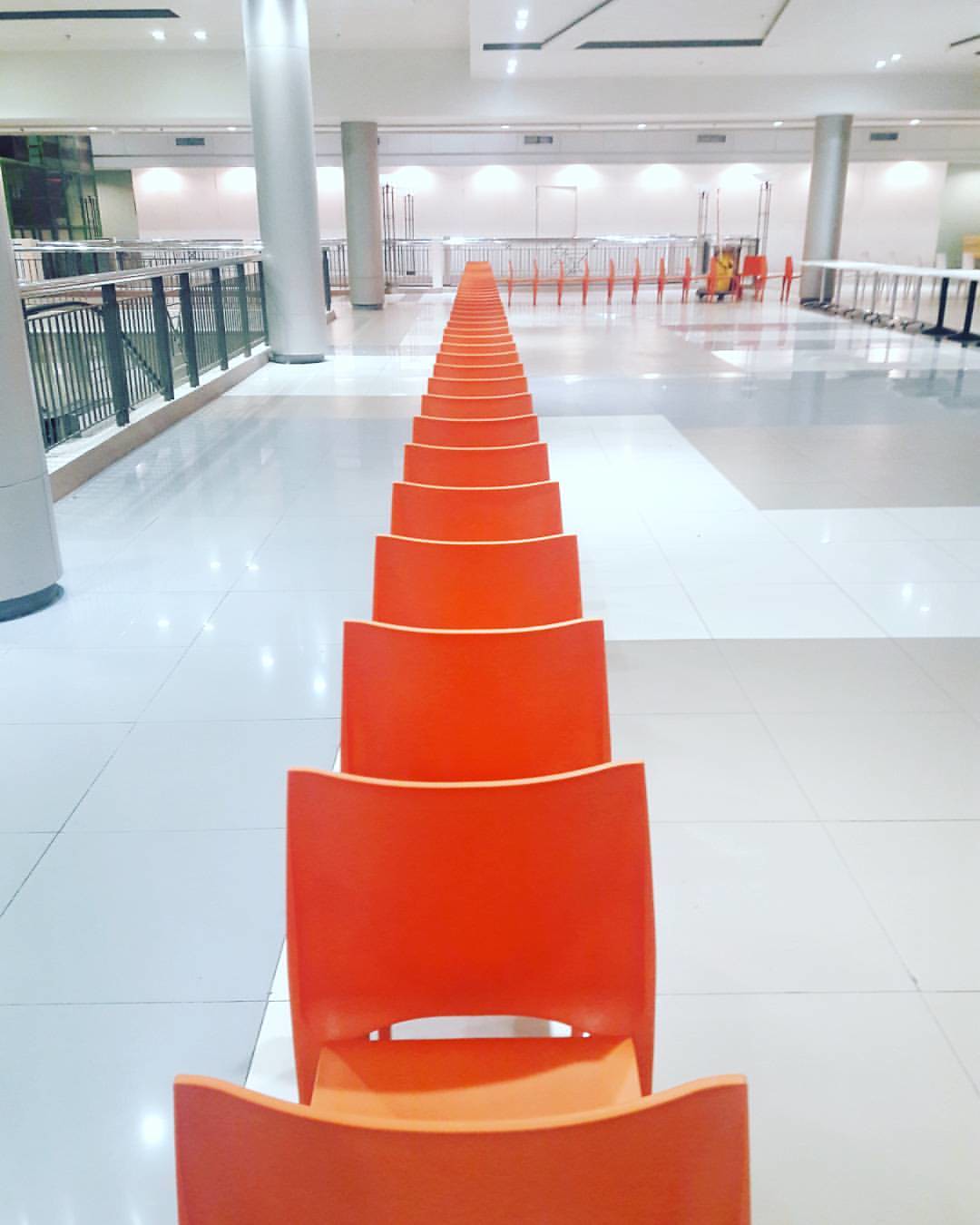This photograph depicts an expansive interior space, likely part of an airport or a large commercial building such as a mall. The scene is characterized by shiny white and gray tiled flooring, interrupted intermittently by large round columns. Central to the image is a long row of bright orange plastic chairs that stretches from the foreground to the distance, eventually turning to the right and continuing out of view. The chairs are neatly arranged one behind the other. 

The left side of the image features black railings, hinting at the presence of a second story vantage point, possibly overlooking a lower level. An escalator is partially visible with its handrail disappearing into the floor, suggesting vertical connectivity within the space. Additionally, a small cart is seen, hinting that it may have been used to place the chairs, although no people are visible in the photograph.

In the background, a white wall with chrome-colored fencing, doors, and several ventilation vents, stands illuminated by numerous spotlights embedded in the ceiling. The columns supporting the structure are spaced equidistantly, adding to the sense of vastness. To the far right, the upper corner reveals what appear to be white tables on either chrome or black pedestals. The overall aesthetic of the space, combined with the architectural elements and the vibrant arrangement of chairs, conveys a modern yet utilitarian environment.